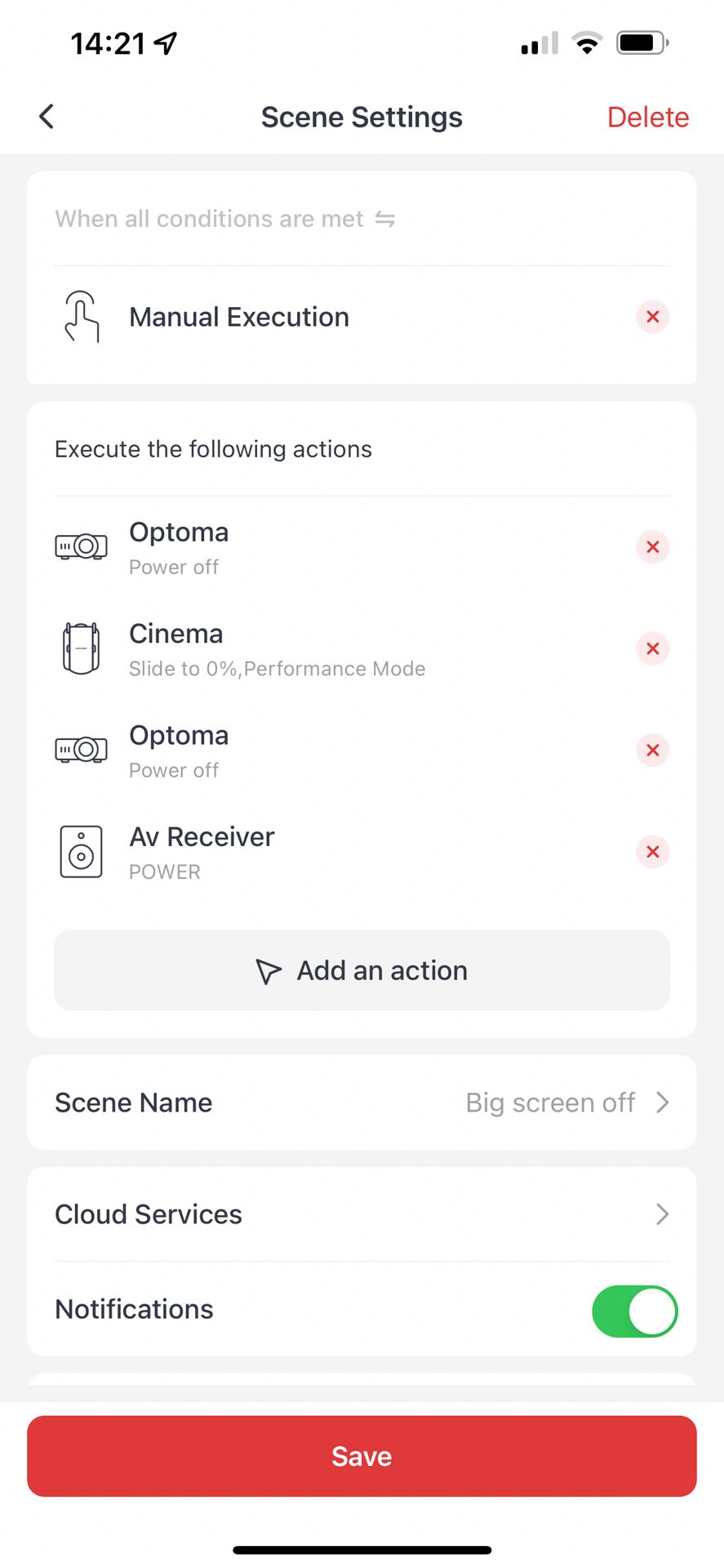The image predominantly features an all-white background. In the top left corner, the time is displayed as 14:21. Adjacent to this, at the top of the screen, there are icons indicating cellular signal strength, Wi-Fi connectivity (represented by a small fan icon), and a battery indicator. 

Centrally positioned, there is a section labeled "Scene Settings." To the right, the word "DELETE" is written in red. The text "When all conditions are met" is displayed prominently, followed by the phrase "Manual Execution," accompanied by a finger-pointing icon. Below this, the instruction "Execute the following actions" is listed.

There are several labeled actions:
1. "Optima" with a "Power Off" command.
2. "Cinema" with "Slide to 0% Performance Mode."
3. "Optima" again with "Power Off."
4. "AV Receiver Power."

Each action is prefixed with small icons. To the right of these actions, there are red X's and additional pink circles.

At the bottom of the action list, there is a button labeled "Add an Action," marked with an upwards arrow icon. Underneath this, a section titled "Scene Name" highlights the term "Big Screen Off." Further down, it indicates that "Cloud Services and Notifications" are enabled, evidenced by a highlighted green button.

Finally, at the very bottom of the image, there is a red, rectangular button labeled "SAVE."